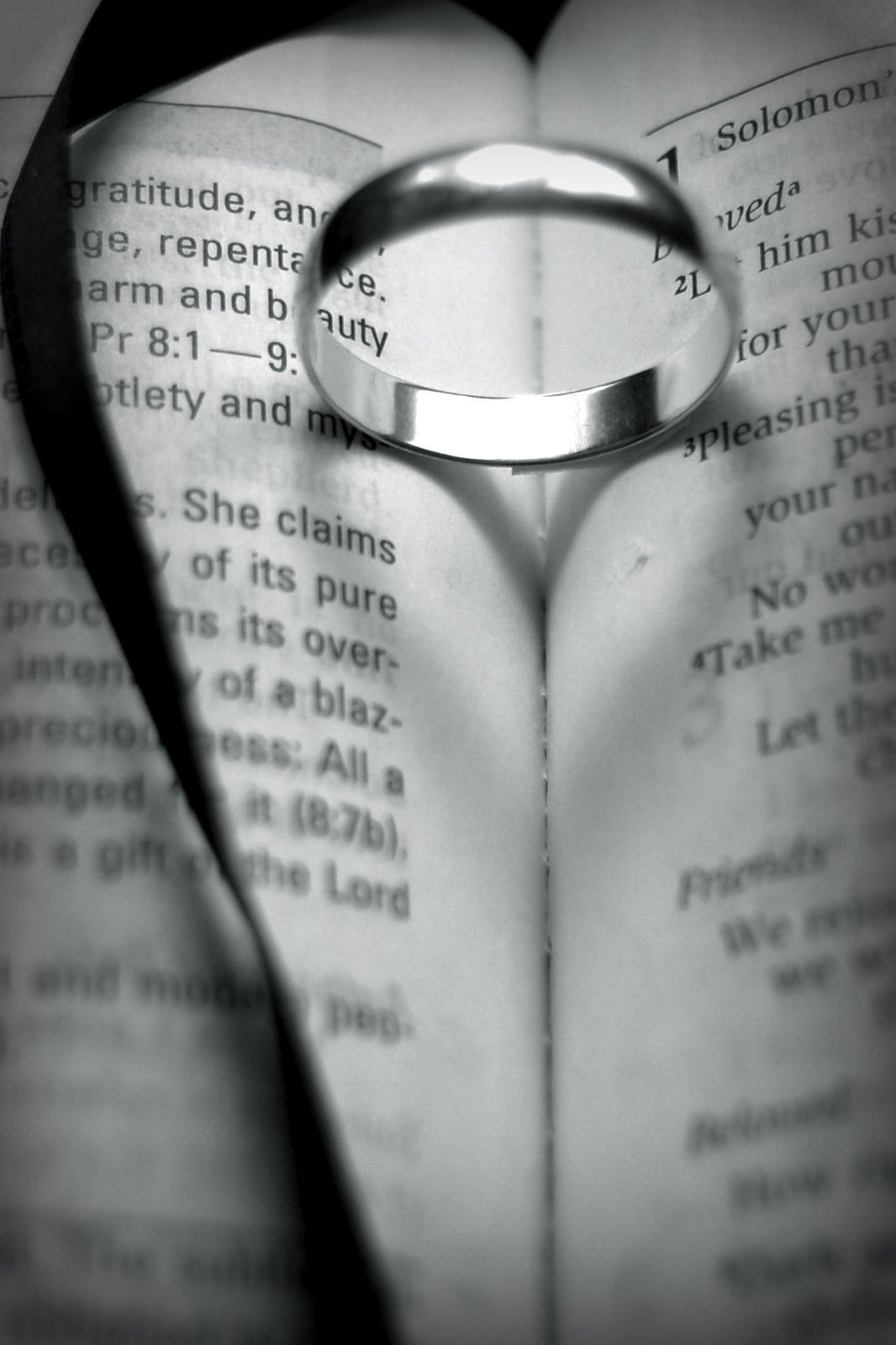This black-and-white photograph captures a serene and contemplative scene of an open book, with the pages spread to the midpoint, revealing the spine running vertically, slightly off-center. Positioned delicately upright within the book's crease is a simple, unmarked silver ring, which seems to bridge the gap between the two pages. Adding to the composition, a black ribbon bookmark trails from the top left corner, cascading diagonally down towards the bottom middle of the image. The text on the book's pages comes into partial focus, offering glimpses of various words such as "gratitude," "repentance," "beauty," and "friends" on the left, along with "Solomon," "pleasing," "take," and "let" on the right. The photograph's focus gradually softens as it moves towards the bottom, creating a delicate contrast in clarity that enhances the meditative quality of the scene.